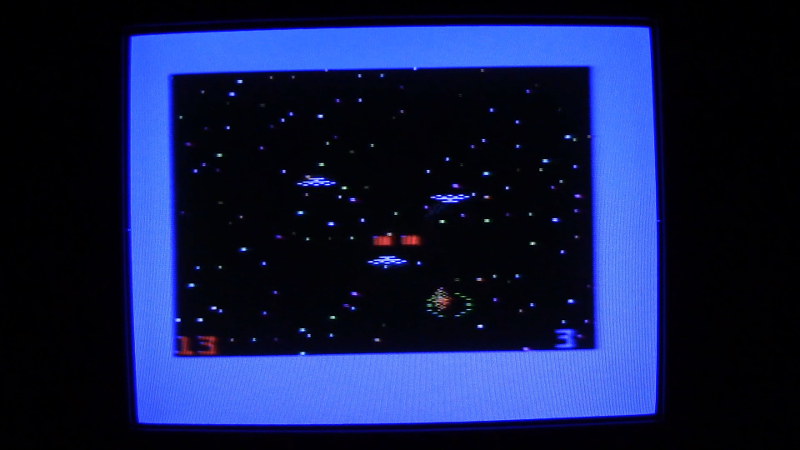A retro video game scene is depicted, reminiscent of classic Nintendo or Atari games. The background is a solid black screen, bordered by a radiant, light blue frame. This border could potentially be the edge of an old computer monitor, possibly appearing white due to a glowing effect. Scattered across the black screen are clusters of white dots, representing stars in the void. A numerical '13' appears in white in the lower left corner, while another '13' in red is positioned in the lower right corner, adjacent to a blue '3'. The central part of the screen showcases three small shapes resembling butterflies, intricately detailed and seemingly in mid-flight. Two red dots are prominently displayed in the center of the screen. Toward the lower right, a formation of yellow dots encircle a larger red dot, creating a striking contrast against the dark background.